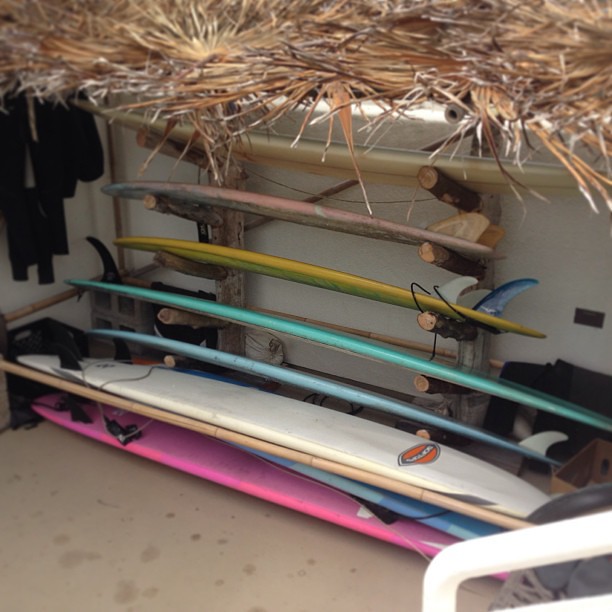The photograph showcases the interior of a surf shop, featuring an array of surfboards displayed on a rustic wooden rack. The rack, which looks homemade, is crafted from logs and pieces of wood. The surfboards are arranged vertically by size, with the longest at the bottom and progressively shorter ones stacked above. The color sequence is noteworthy: at the bottom is a pink surfboard, followed by a white one with an orange and black logo, then a faded light blue board, a teal one, a yellow one, and finally a light pink surfboard. The setting has a relaxed, beach-inspired vibe with a tan stone or cement floor and white walls. At the top of the display, a thatched, tiki bar-like roof hangs along with some brown, ruffled leaves or dead plants. Additionally, a black coat or surf suit is hanging on the top left of the white wall, adding to the casual, coastal decor.